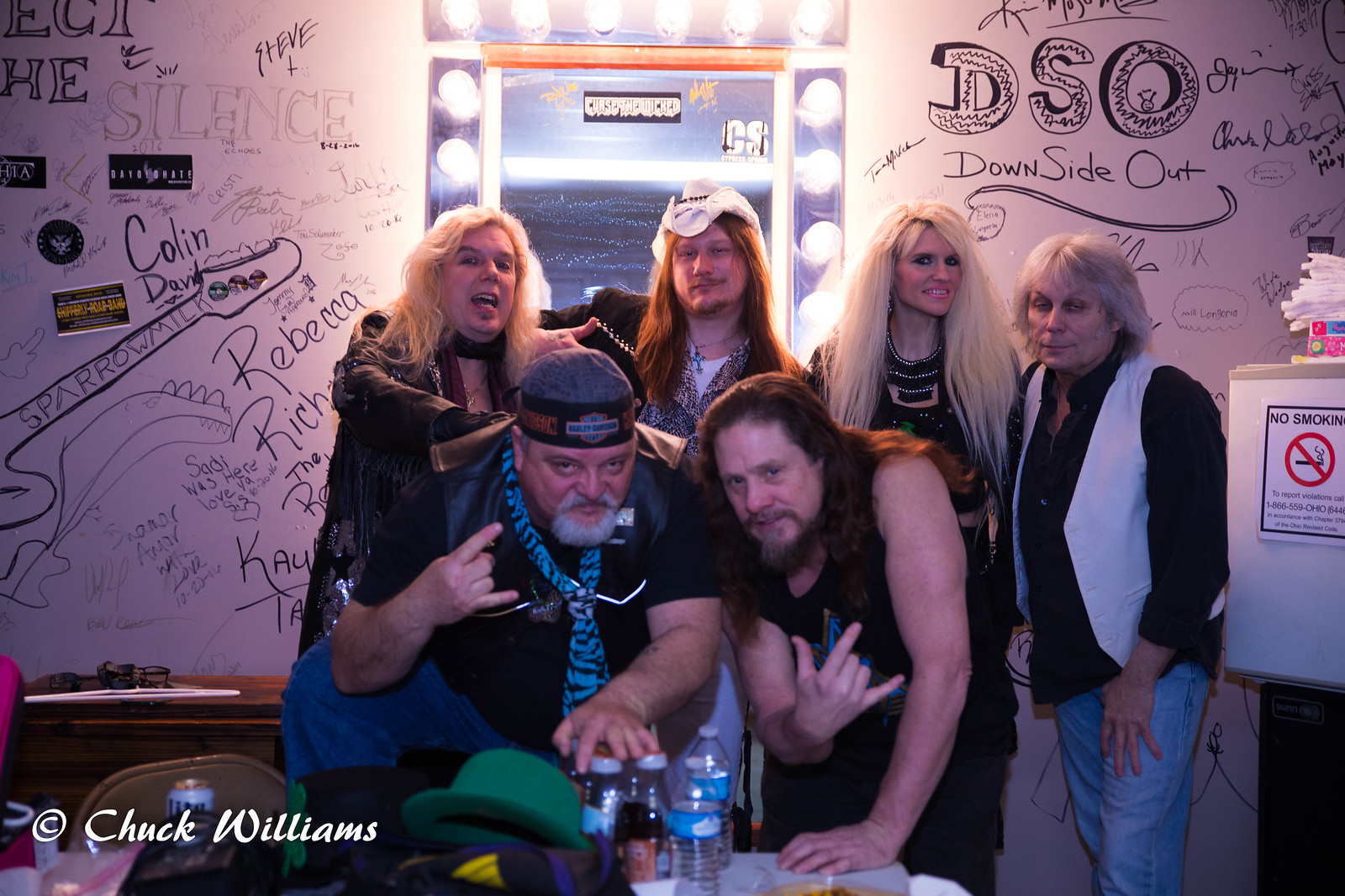This photograph captures six individuals in what appears to be a dressing room, evident from a large mirror framed with spotlight bulbs behind them. The group, possibly members of a heavy metal rock band, exudes a tough, biker-like aesthetic, dressed in leather, biker gear, and tank tops. Their long hair varies from dark to blonde, with some wearing distinctive accessories such as cowboy hats. In the background, graffiti and signatures cover the white or dry erase walls, adding a grungy feel to the setting. Four people stand in the back, including two men with long blonde and brown hair, a woman with long blonde hair, and an older man with shorter gray hair, dressed in jeans, a black button-up shirt, and a white vest. Two men in the front lean over a cluttered table, making hand symbols reminiscent of the "Hang Ten" gesture. The table is scattered with water bottles, clothing items, and a green hat. In the lower left corner of the image, the text "Chuck Williams" signifies the photographer's copyright. The scene, rich in detail, presents a vivid snapshot of a possibly intense and lively pre-performance moment.